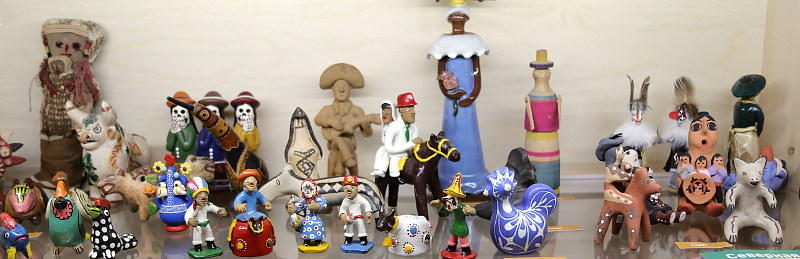The image depicts a vibrant collection of approximately 40 intricately designed and colorful porcelain figurines arranged on a glass shelf. The backdrop features a beige wall with white molding at the bottom, adding a subtle contrast to the vivid display. Among the figurines, there are several noticeable themes and characters: some are decorated with different faces and bows, while others appear more whimsical and creative. Notable among them are three skeleton figurines donning top hats, which might hint at cultural influences, possibly Mexican. There's also an array of animals, including a bull, chickens, and a rooster adorned with white designs. One intriguing piece shows a figure riding a black horse, dressed as a doctor with a red hat, and another features a musician wearing a sombrero and playing a guitar, albeit unpainted. Additionally, a gray hyena with distinctive black stripes on its arms and legs adds to the diverse and imaginative ensemble. Skulls can be seen subtly in the background, contributing to the eclectic and artistic display.